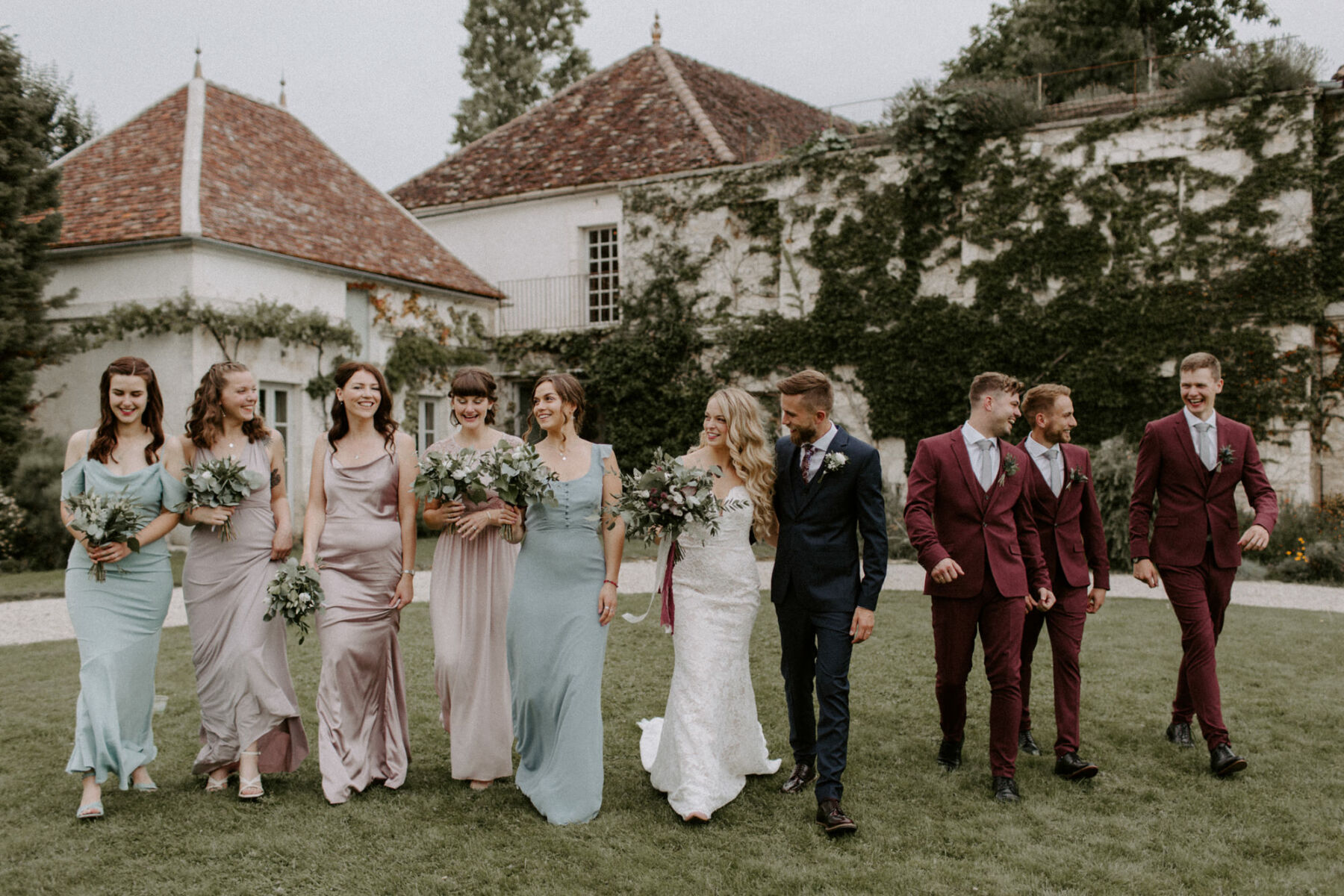The image captures a picturesque wedding scene set on the manicured lawn of a grand manor house adorned with overgrown ivy clinging to its stucco walls. The house, characterized by its red clay-tiled roof, provides a majestic backdrop to the bridal party. The overcast sky lends a soft, diffused light to the ensemble.

In the center of the photograph stand the bride and groom. The bride, with her long, curled hair cascading over her shoulders, is radiant in a strapless white gown with a sweetheart neckline, holding a large, lush bouquet. The groom, sporting dark hair and a neatly groomed beard, wears a dark suit with a boutonniere and a straight tie tucked into his vest. To their sides are the bridesmaids and groomsmen.

The five bridesmaids are arranged on either side, wearing dresses in shades of sage green and light plum, each in a different style. Their coordinated yet unique looks are completed with matching bouquets. All the bridesmaids are brunettes, with varying hairstyles—some with their hair down, others with it pulled back. The groom’s party, comprising three groomsmen, are dressed in dark maroon suits with white shirts, dark vests, and coordinated ties. Each groomsman sports a boutonniere, and they are captured mid-conversation, adding a touch of candid joy to the scene.

Behind the group, a curving road and a sidewalk path are visible, adding depth and context to the photograph, suggesting that the manor house could be either behind or in front of the grassy area where they stand.

The overall setting is both grand and intimate, showcasing not just the detailed attire of the wedding party but also the historical elegance of the manor house and its idyllic surroundings.